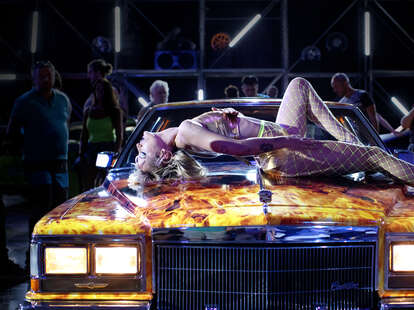This is an image from what appears to be a photo shoot featuring a young, blonde woman posing seductively on the hood of a flashy Cadillac from the 1980s or early 1990s. The hood and front bumper of the car are strikingly painted with vivid yellow and red flames. The woman, dressed provocatively, is positioned with her head and bottom touching the hood, one leg lifted so her heel rests on the car. The headlights of the car are illuminated, contributing to the dramatic scene. In the background, several people are visible; some are watching, while others are talking amongst themselves. Overhead lights shine down on the scene, enhancing the photo shoot's ambiance. There are also shelves in the background, possibly holding a ghetto blaster or other items, adding to the setting's detail.